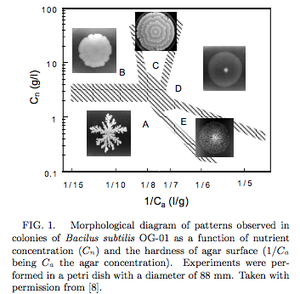The image is a detailed morphological diagram of patterns observed in colonies of Bacillus subtilis OG-01, focusing on the nutrient concentration \(C_n\) and the hardness of the agar surface \(1/C_n\), with experiments conducted in a Petri dish with a diameter of 88 mm. The diagram is set against a white background and is enclosed in a rectangular frame with a black border. The x-axis is labeled \(1/C_n\) (with units possibly in \(l/g\)) ranging from \(1/16\) to \(1/5\), while the y-axis is labeled \(C_n\) (with units likely in \(g/l\)) ranging from 0.1 at the bottom to 100 at the top. Inside the rectangle, there are five squares labeled A, B, C, D, and E, each containing black and white images depicting the bacterial colony patterns. Below the rectangle, there is descriptive text in black: "FIG-1: Morphological diagram of patterns observed in colonies of Bacillus subtilis OG-01 as a function of nutrient concentration \(C_n\) and the hardness of the agar surface \(1/C_n\), being \(C_n\) the agar concentration. Experiments were performed in a Petri dish with a diameter of 88 mm, taken with permission from [source]."